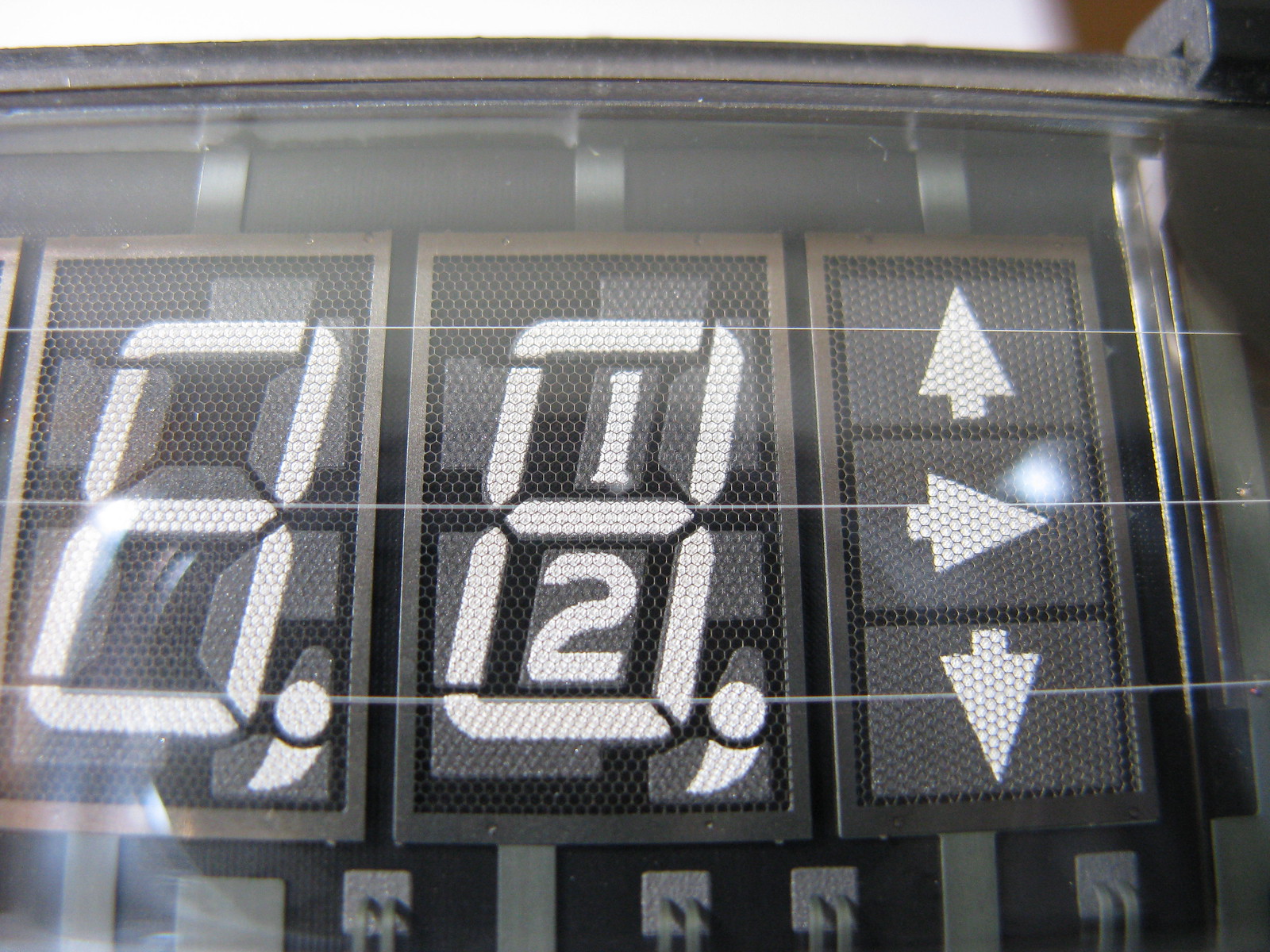The image appears to be a highly zoomed-in view of a digital display, reminiscent of those found on gas pumps or alarm clocks. The focal point of the image is three distinct sections. On the left, two sets of numeric displays show digits that can increase or decrease; these numbers are displayed on a white background. The digits on the first display appear to show the number "88," while the second display portrays an intriguing mix of numbers and symbols: an "8" at the top, a "1" in the middle, and a "2" at the bottom. On the right side of the image, there are arrow indicators, likely for navigation or adjustment purposes. The backdrop is a dark gray and black arrangement, featuring rectangular shapes, providing contrast to the bright numerical displays. The entire display is encased in a bronze or brown-colored border, adding a slightly vintage or industrial feel to the scene. The extreme close-up nature of the photograph makes it challenging to discern the exact type of machine or device, leaving it open to interpretation.